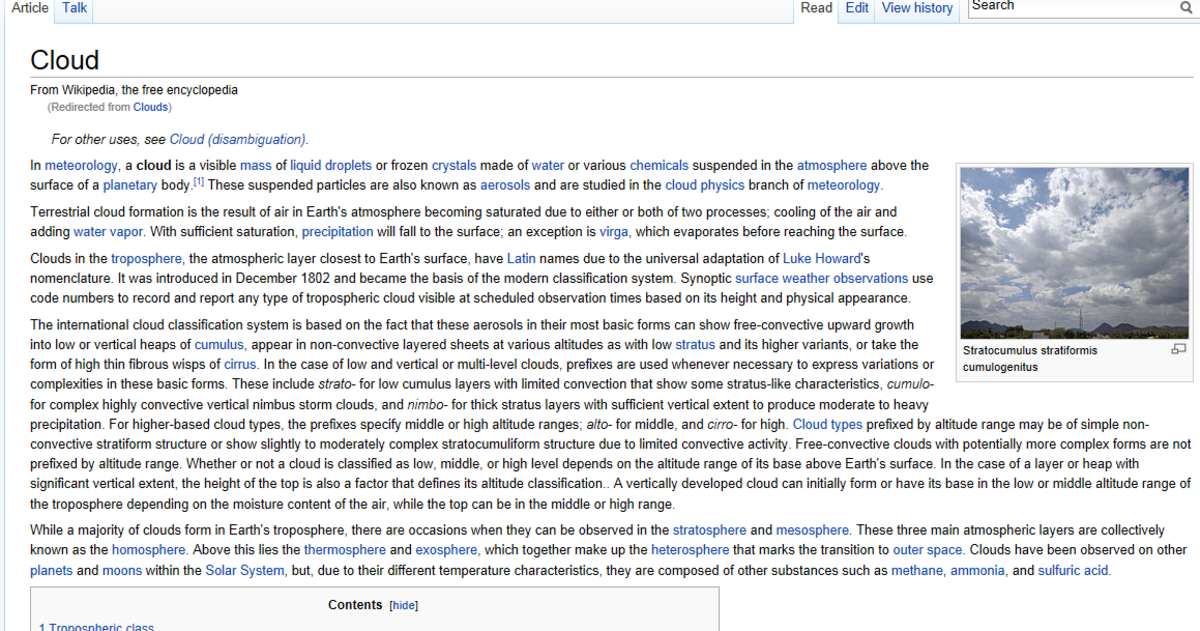Clouds, as defined in meteorology, are visible masses composed of liquid droplets or frozen crystals of water, along with various chemicals, suspended in the atmosphere above a planetary surface. These suspended particles, known as aerosols, are studied within the cloud physics branch of meteorology. On Earth, clouds form when air in the atmosphere becomes saturated, either by cooling or by the addition of water vapor. This saturation can result in precipitation, which may evaporate before reaching the surface. 

In the Earth's troposphere, cloud formation is influenced by atmospheric dynamics and is characterized based on height and physical appearance. The international cloud classification system categorizes clouds into various types, such as cumulus (heaped, low-level clouds), stratus (layered sheets), and cirrus (high, thin, fibrous clouds). In cases where clouds span multiple levels or exhibit significant vertical development, additional prefixes help describe their complex structures. This classification aids meteorologists in observing, recording, and predicting weather patterns. Using standardized code numbers, they report these observations at set intervals, contributing to a comprehensive understanding of atmospheric conditions.